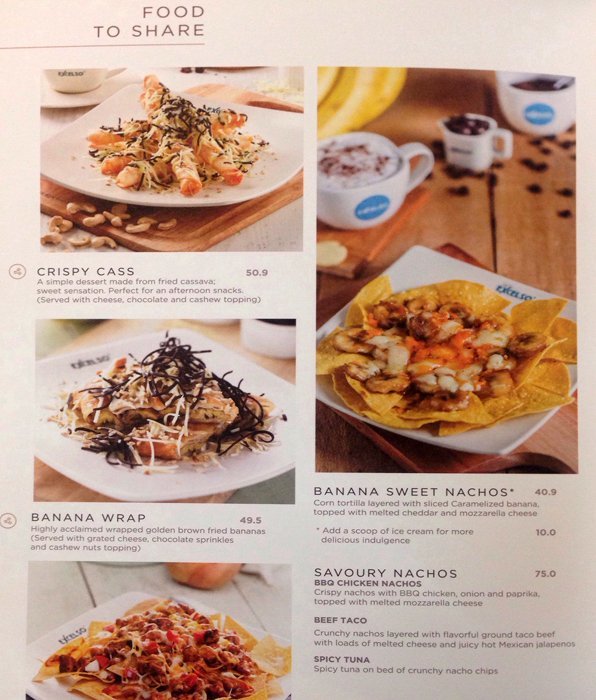The image showcases a restaurant menu with a white background, featuring four different food items prominently displayed with images and descriptions. At the very top of the menu, the heading "Food to Share" is clearly visible. 

The topmost item on the left is "Krispy Kass," a simple dessert made from fried cassava, described as a sweet sensation perfect for an afternoon snack, served with cheese, chocolate, and cashew topping. Below "Krispy Kass" is an image of a "Banana Wrap," featuring highly acclaimed golden brown fried bananas, served with grated cheese, chocolate sprinkles, and cashew nuts topping. 

To the right of the "Banana Wrap" image is a picture of "Banana Sweet Nachos," comprising layers of corn tortilla and sliced caramelized bananas, adorned with melted cheddar and mozzarella cheese. 

The bottom left of the menu displays another nacho-style dish with a wooden table setting. Although less clear, the description to its right identifies it as "Savory Nachos," offering three variations: Barbecue Chicken Nachos, Beef Taco Nachos, and Spicy Tuna Nachos. 

This detailed layout and vivid imagery aim to entice customers to share and enjoy these delectable offerings.